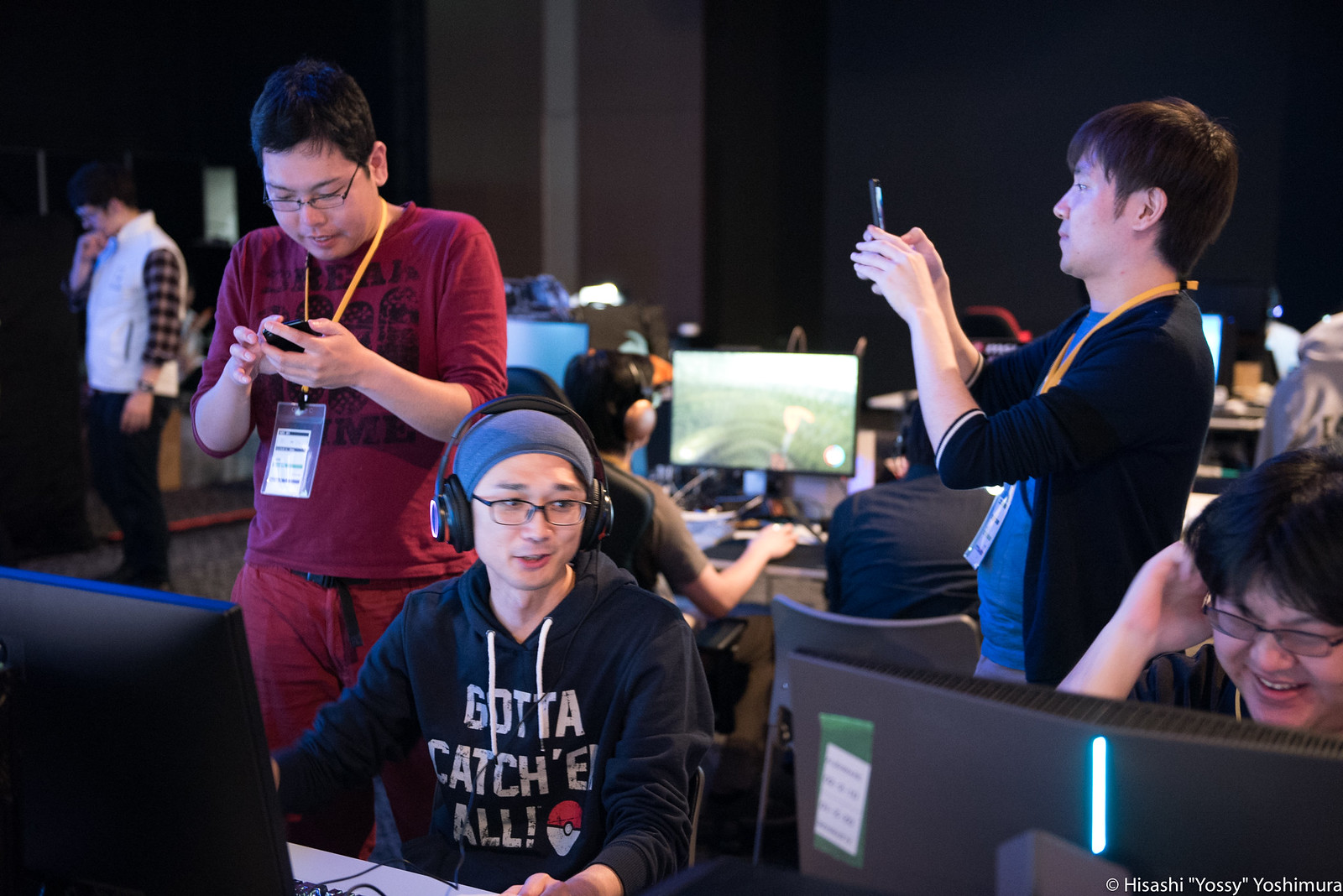In a bustling room filled with numerous computer screens, several individuals are engrossed in their activities. At the center-left, slightly towards the bottom, a person with a blue scarf on their head is seated, wearing black headphones and glasses. They are looking downward and don a hoodie with the text "Gotta catch a haul" written on the chest, accented with white strings. Just behind them to the left, another individual wearing an amber-colored shirt and shorts stands, holding a phone to their chest. A yellow lanyard with a clear plastic card dangles from their neck. They have black hair and glasses and are absorbed in their phone. To the right side, a man dressed in a black shirt with sleeves rolled just below his elbows is pointing a phone directly toward the aforementioned person. He also wears a yellow lanyard around his neck and sports black hair. The room features a dark black wall in the background, punctuated with a few gray lines, and numerous people are both standing and seated, engaged with their screens. A person in the back stands out in red attire, and another person in a white dress appears to be talking on the phone. One particular computer screen in the center displays green colors and is marked with the copyright, "HISASHI 'YASI' YASHIMURA" at the bottom right. The overall ambiance suggests a dynamic conference or collaborative event, with participants interacting with both digital devices and each other.